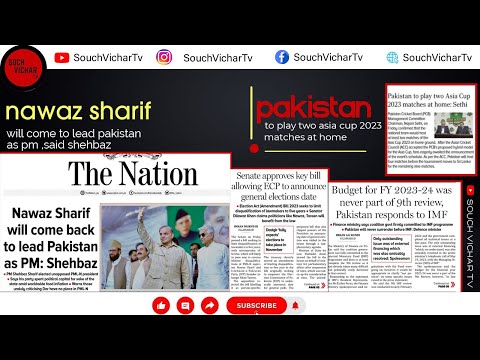The image showcases a news website, possibly from Pakistan, featuring multiple news articles and newspaper clippings. Central to the page, a headline reads "Nawaz Sharif will come back to lead Pakistan as PM, says Shabazz," accompanied by a picture of Nawaz Sharif standing on a stage, waving to a crowd, with several aides around him. On the right side, another headline announces "Pakistan to play two Asia Cup 2023 matches at home." The website has a clean layout with a white banner at the top that includes links to their social media platforms, such as YouTube, Instagram, Facebook, and another unrecognized logo. The site appears to be dedicated to news, emphasizing its journalistic focus with various clippings and articles presented prominently.